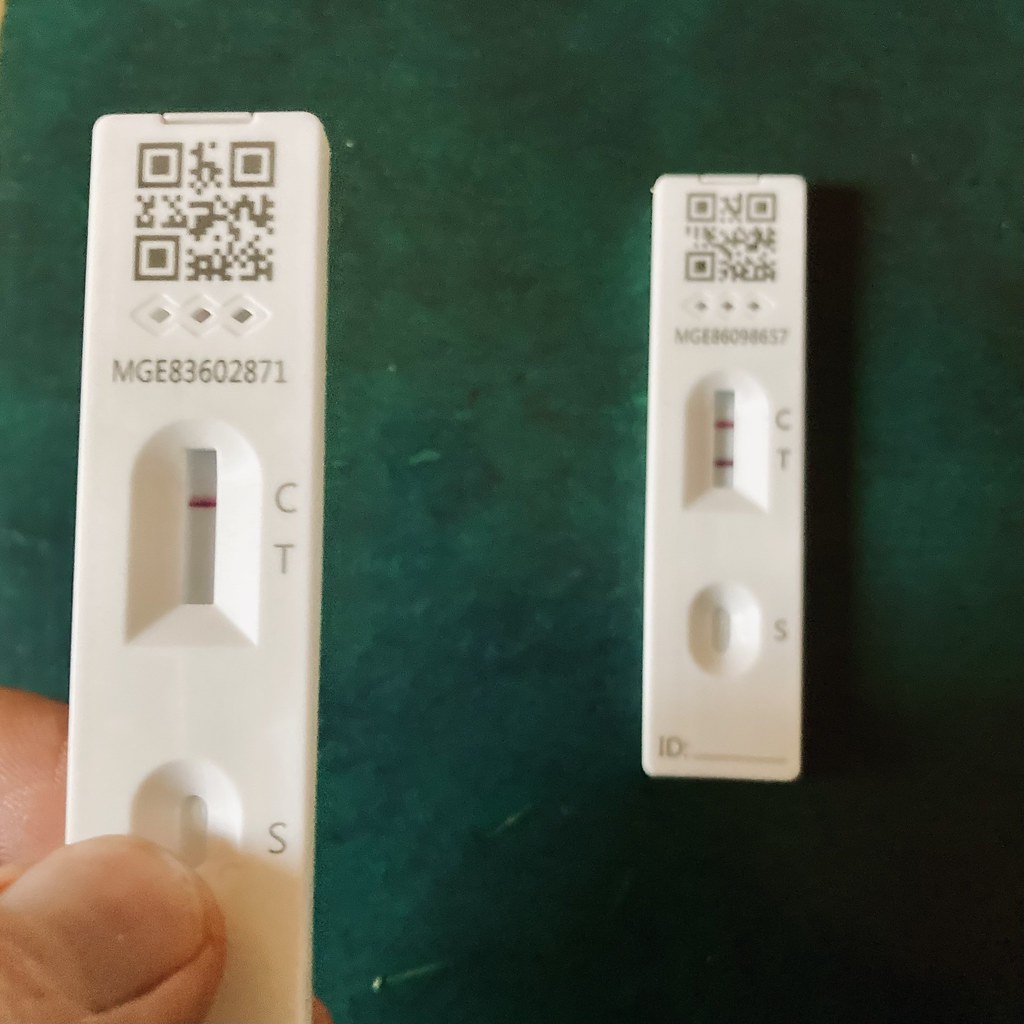The image features a green marbled texture in the background, which forms the surface upon which the objects rest. The focal point of the image is two COVID-19 test kits, albeit somewhat blurry. The test kit on the right is in direct contact with the green surface and appears less focused. At the top of this test kit is a QR code accompanied by three small diamonds, likely serving as indicators. The code "MGE360-95657" is visible, which is presumably an identifier for the COVID-19 test. Both the 'C' (control) and 'T' (test) markers on this kit are marked in dark red, suggesting a positive result. The sample area, located at the bottom part of the kit, features an oblong circle with a smaller pill-shaped section marked with an 'S' next to it, followed by the number '10' and some other indistinct text.

In contrast, the second test kit in the image is held by someone's hand and is more in focus. Identified by the code "MGE83602871," this kit shows a red 'C' marker, but the 'T' marker remains uncolored, indicating either a negative result or an incomplete test. The person's thumb is positioned on the lower section of the kit, near the sample application area, mirroring the design of the other kit. The clear distinction between the two kits, in terms of focus and results, adds a layer of depth to the narrative of the image.